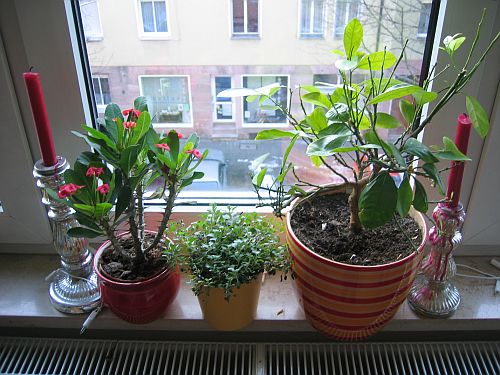The photograph captures a view from a second or third-story apartment window, likely in an urban area resembling Brooklyn, New York. The large square window, devoid of any dividers or wood panes, offers an unobstructed view of a red-brick apartment building with a white upper story directly across the street. Below the window inside the apartment, a wooden shelf holds three distinct clay pots with lush greenery. On the left, there’s a Crown of Thorns plant with waxy green leaves and tiny red flowers in a round, belly-shaped red pot. The center pot, a straight-sided yellow ceramic one, contains what appears to be thyme or another herb. The largest pot on the right, adorned with red, white, and yellow stripes, holds a philodendron-style plant or a money tree. This arrangement is flanked symmetrically by two silver candlesticks with burned red taper candles. The interior detail, including what seems to be a radiator beneath the window, adds to the cozy, urban apartment ambiance.